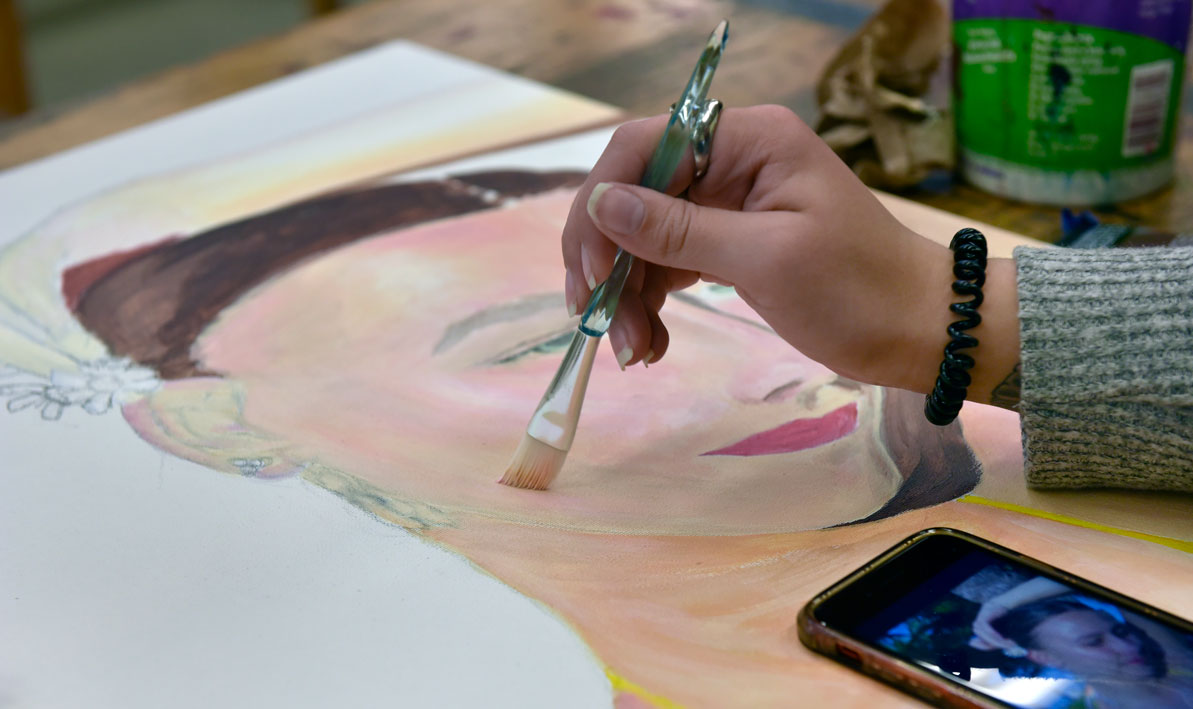In the image, a person, likely a woman, is seen painting a portrait of another woman on a white canvas. The painter's hand, adorned with a black bracelet and possibly a tattoo on the wrist, holds a paintbrush poised on the canvas. The hand, emerging from a long-sleeve shirt or sweater, is captured mid-stroke as the brush traces the contours of the subject's cheek. The portrait on the canvas depicts a Caucasian woman with brown hair partly covering her face, pink lipstick, and green eyes, along with a small white flower near her ear. The painting, still in progress, exhibits soft, gentle hues of pinks and beiges.

In front of the painter, an iPhone displays the reference image of the woman's face, mirroring the features being painted. The entire scene is set on a round, wooden table scattered with painting supplies. The atmosphere suggests a moment of focused creativity, with the painter intricately detailing the woman’s likeness from the digital reference on her phone.